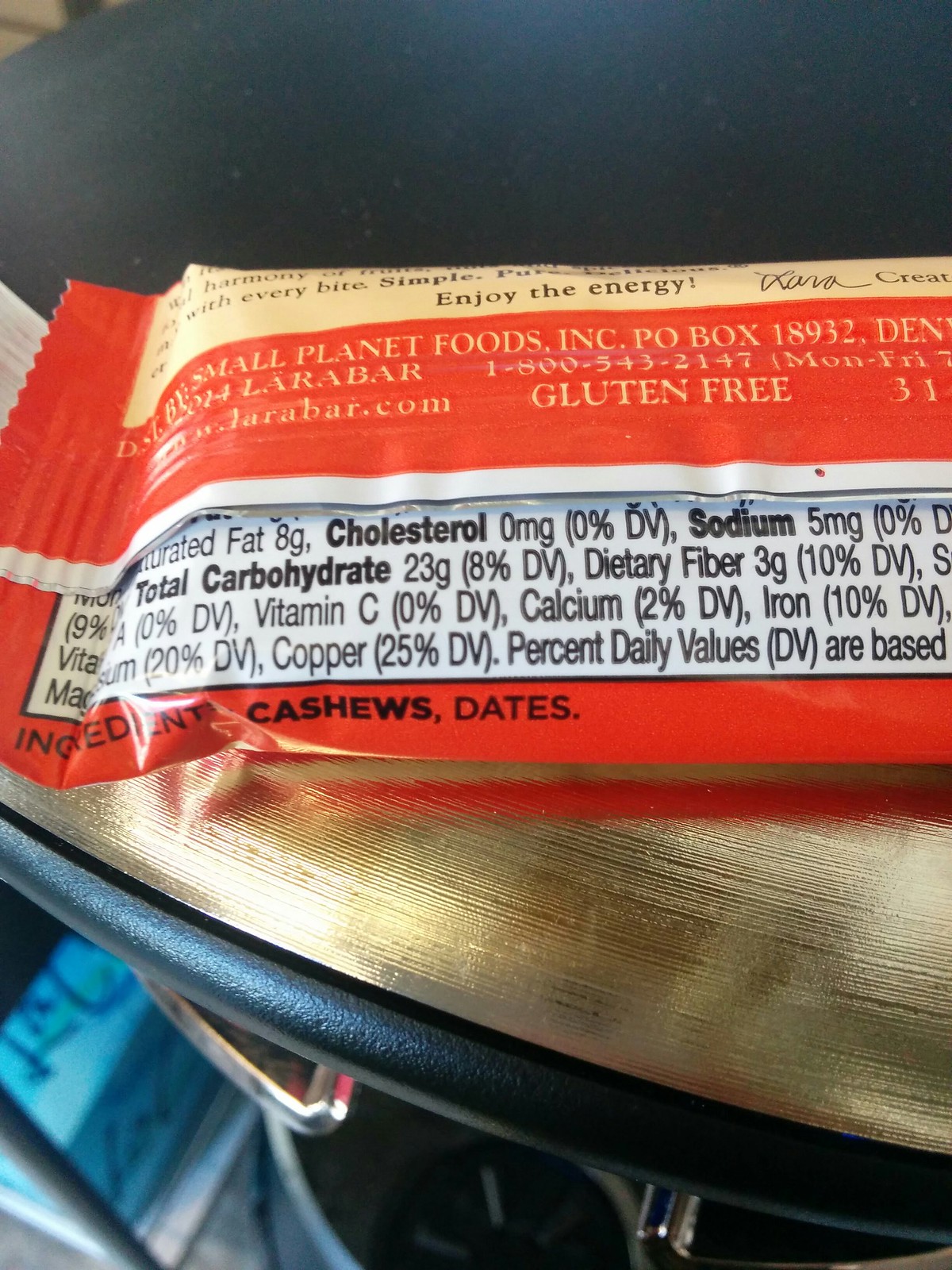This is a close-up color photograph depicting approximately half of an energy bar called a Larabar, packaged in an orange wrapper. The top portion of the package features black text on a yellow background that reads "Enjoy the Energy." Below this, there is a white text on an orange background which includes the name "Small Planet Foods Incorporated" and a P.O. Box 18932. Although partially obscured, a website is also present. Notably, the bar is labeled gluten-free. At the lower part of the wrapper, black text on a white background lists nutritional facts and ingredients like cashews and dates, alongside measurements for cholesterol, sodium, carbohydrates, dietary fiber, calcium (2% DV), iron (10% DV), copper (25% DV), and vitamin content (20% DV). The bar is placed on a golden-colored surface tray that appears etched and features a metallic blue rim. Below the tray, steely-looking legs are visible on a bluish floor, with the top of the image fading into blackness.